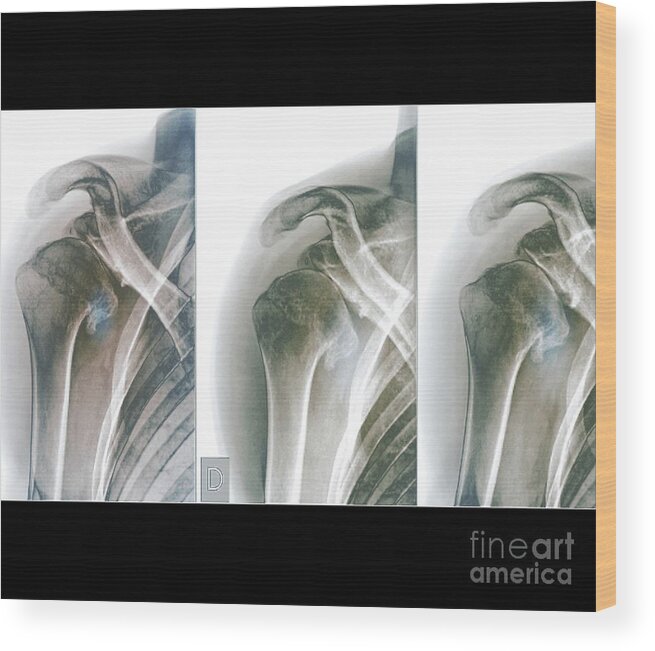The image depicts a series of three detailed 3D color illustrations of an x-ray of a human shoulder, arranged in a side-by-side portrait orientation within a landscape frame. Each illustration presents a side view of the shoulder's interior, showcasing the ribs, musculature, and underlying bone structure beneath the skin. The sequence of images progresses from left to right, with the leftmost illustration showing the most severe rupture at the top joint of the shoulder bone. The central image reveals a slightly ameliorated condition, while the rightmost illustration displays the shoulder bone fully intact, indicating a healing process. The images are bordered by horizontal black stripes at the top and bottom, with a pink-beige border on the sides that gives the appearance of a wrapped canvas, enhanced by a woodgrain texture on the sides. At the bottom right corner of the illustration, the text "Fine Art America" appears in semi-transparent white.